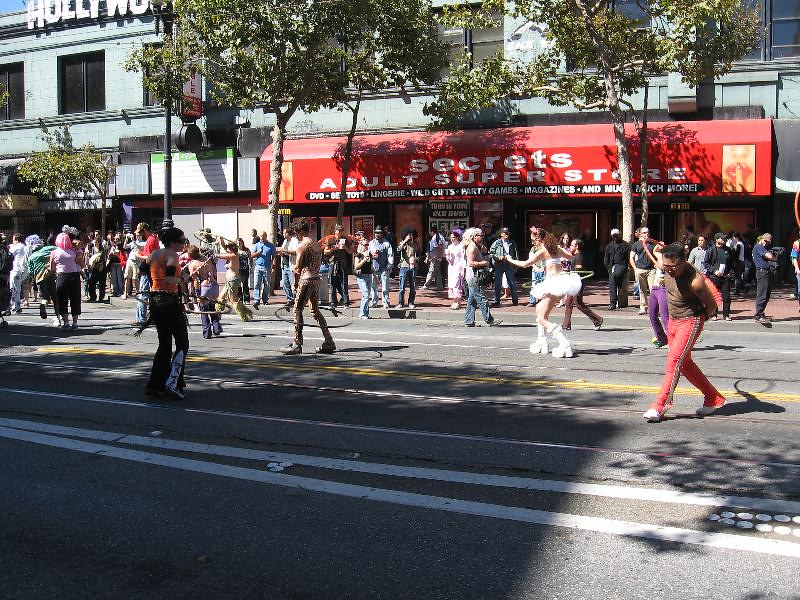The photograph captures a vibrant street parade on a sunny day. The scene is bustling with people dressed in intriguing and diverse costumes, ranging from no tops to tights, and even hula hoops. A standout costume includes a woman in a white tutu and tall platform shoes, while another individual appears to be juggling a hula hoop around their knees. The parade passes in front of a store with a prominent awning that reads, "Secrets Adult Superstore," advertising an array of items like DVDs, toys, lingerie, wild gifts, party games, and magazines. The sidewalk is lined with spectators and shaded by trees. In the upper left corner, a building with a sign mimicking Hollywood's iconic lettering hints that this could be in a downtown area, possibly Hollywood. The atmosphere is lively and celebratory, with a mixture of performers and onlookers adding to the festive environment.